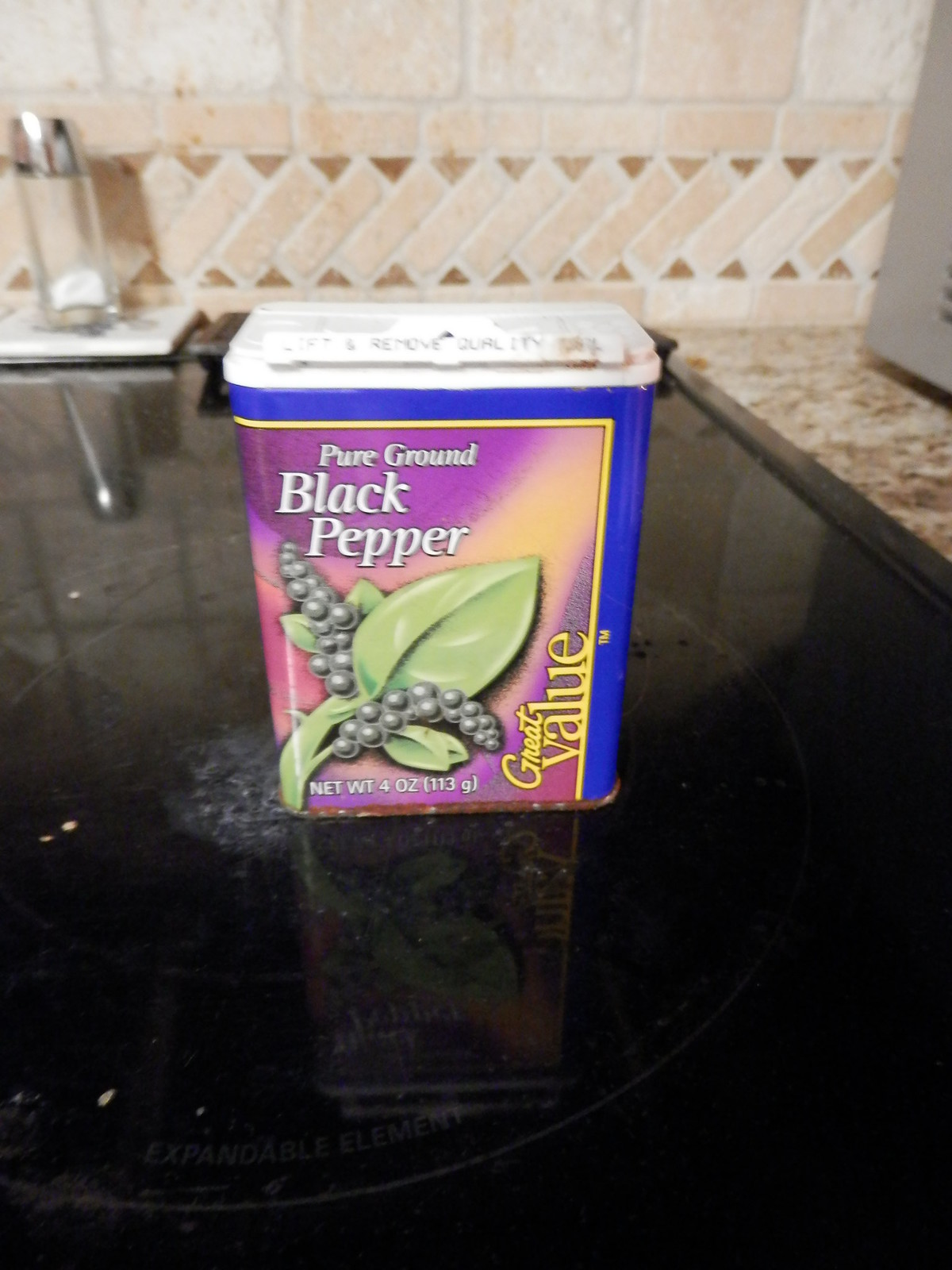This descriptive caption synthesizes the information provided:

---

The image showcases a small container of pure ground black pepper from the Great Value brand. The container features a blue background with a yellow line stating "Great Value" against a purplish backdrop adorned with illustrations of pepper leaves and berries. The label details the net weight as 4 ounces (113 grams). The top of the canister is white plastic, while the bottom appears slightly rusty. The container is placed on a black, glass-top stove, which has an expandable element. Adjacent to the stove is a nearly empty glass salt shaker with a silver top. The background reveals a kitchen with a mottled brown, tan, and white tile backsplash and countertop.